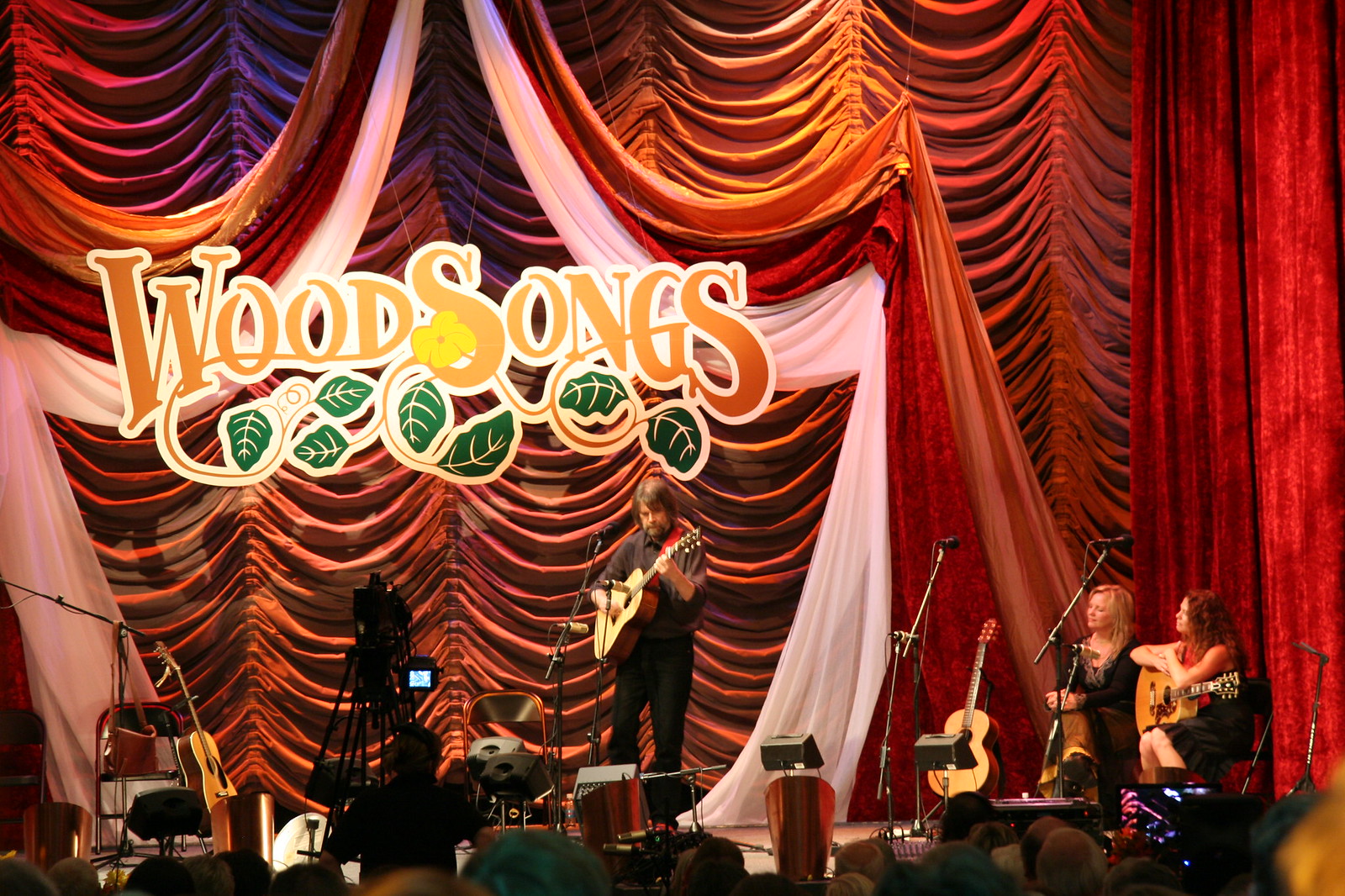The photograph captures a musical presentation on stage, with a significant focus on a man playing an acoustic wooden guitar at the center. He stands in front of a microphone, looking down as he strums his instrument, while a camera to his left records his performance. Directly behind him, a large banner reading "Wood Songs" hangs suspended from the ceiling, adorned with green leaves underneath the text. Flanking the performer on the right side of the stage are two seated women; one of them, positioned furthest to the right, holds an acoustic guitar on her lap, although neither are currently performing. Both women have microphones in front of them, but these are positioned too high for use. The stage is framed by immense orange, white, and pink curtains, dramatically pulled open to reveal an additional set of orange curtains in the background. The heads of numerous audience members are visible at the bottom of the image, emphasizing the event's live and communal atmosphere.